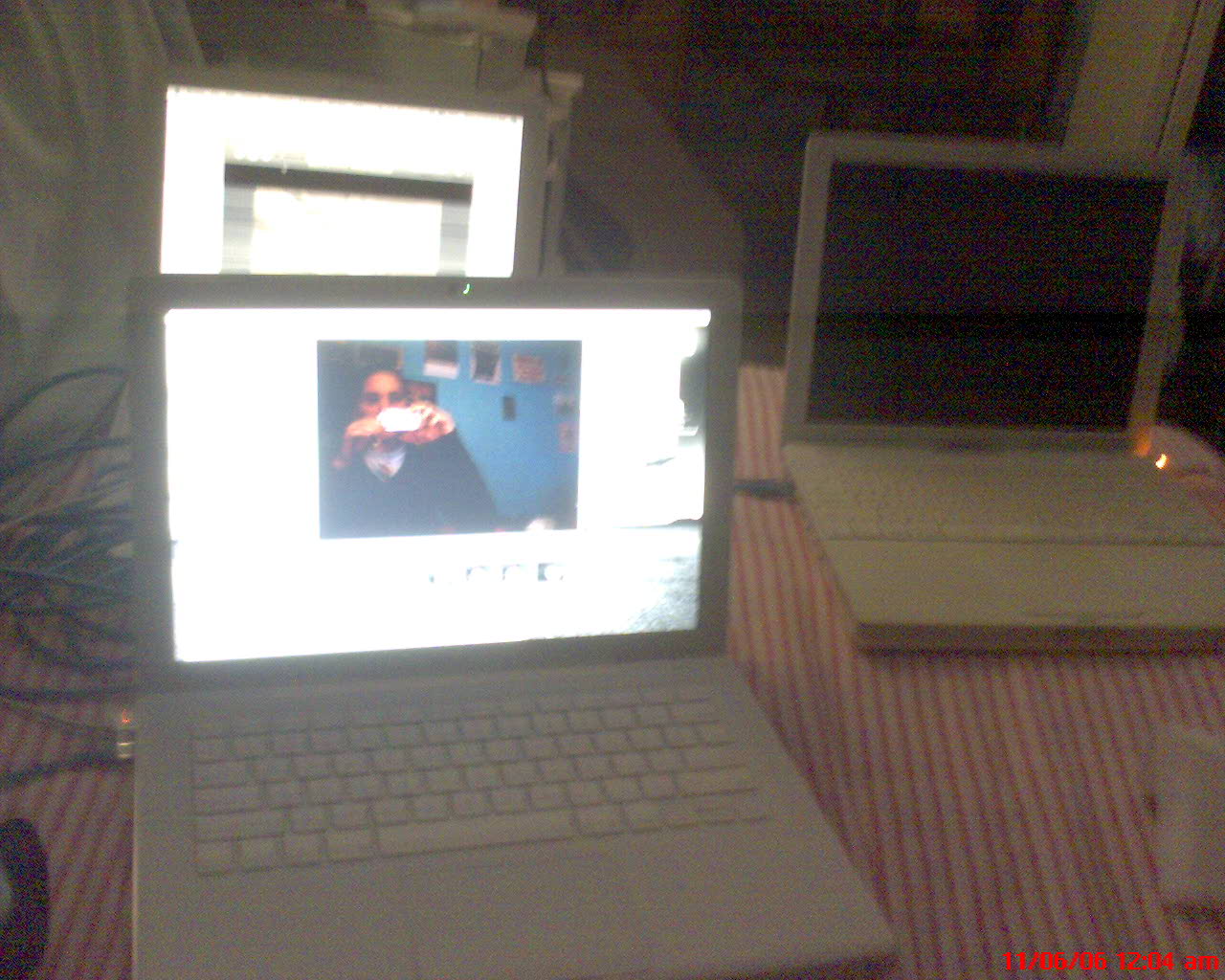The image depicts a very retro scene featuring three off-white, blocky laptops, characterized by their older, thicker designs compared to modern laptops. Positioned on a red and white striped tablecloth, the photo is low-resolution and grainy, further emphasizing its dated aesthetic. In the bottom right-hand corner, a timestamp in red text marks the photograph as taken on 11.06.06 at 12.04 AM. 

In the foreground, two laptops appear prominently. The left laptop's screen glows brightly, nearly blown out, with a distinct image of a woman holding a camera, capturing a selfie against a blue wall adorned with miscellaneous pictures. Directly behind it, the second laptop's screen also illuminates with a bright light and a black square object on a white background. To the right, a third laptop remains open but with a dark, unlit screen, indicating it is either off or in sleep mode. Visible cables and an external mouse hint at the practical use of these devices, despite their now-antiquated appearance.